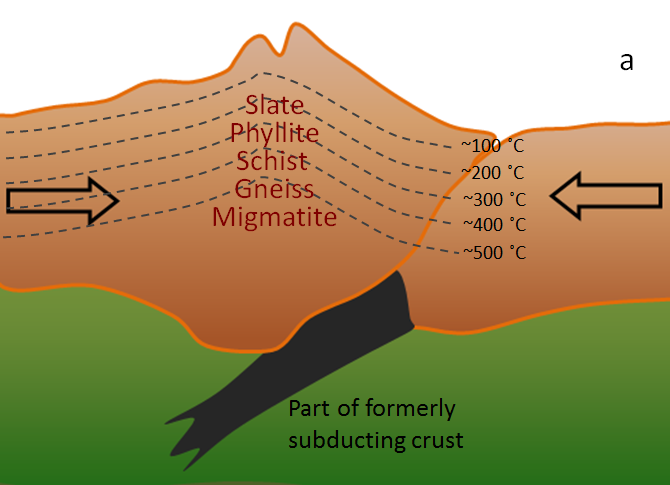This detailed scientific illustration labeled "A" represents a cross-section of different parts of the Earth's crust, specifically at a tectonic plate boundary. The diagram features a ridged landscape at the top and delineates various crust layers from top to bottom: slate, phyllite, schist, gneiss, and migmatite. Each layer is labeled with temperature designations increasing from approximately 100°C at the slate layer up to 500°C at the migmatite layer, shown in red writing. In the green bottom section of the illustration, labeled as "part of formerly subducting crust," a black chunk extends upwards into the orange area above, resembling a gloved hand in shape. This part illustrates the subducted crust that has maneuvered below another plate. Large black arrows on either side of the diagram indicate the direction of the tectonic forces, with both arrows pointing towards each other, demonstrating the process of subduction where one tectonic plate moves beneath another.